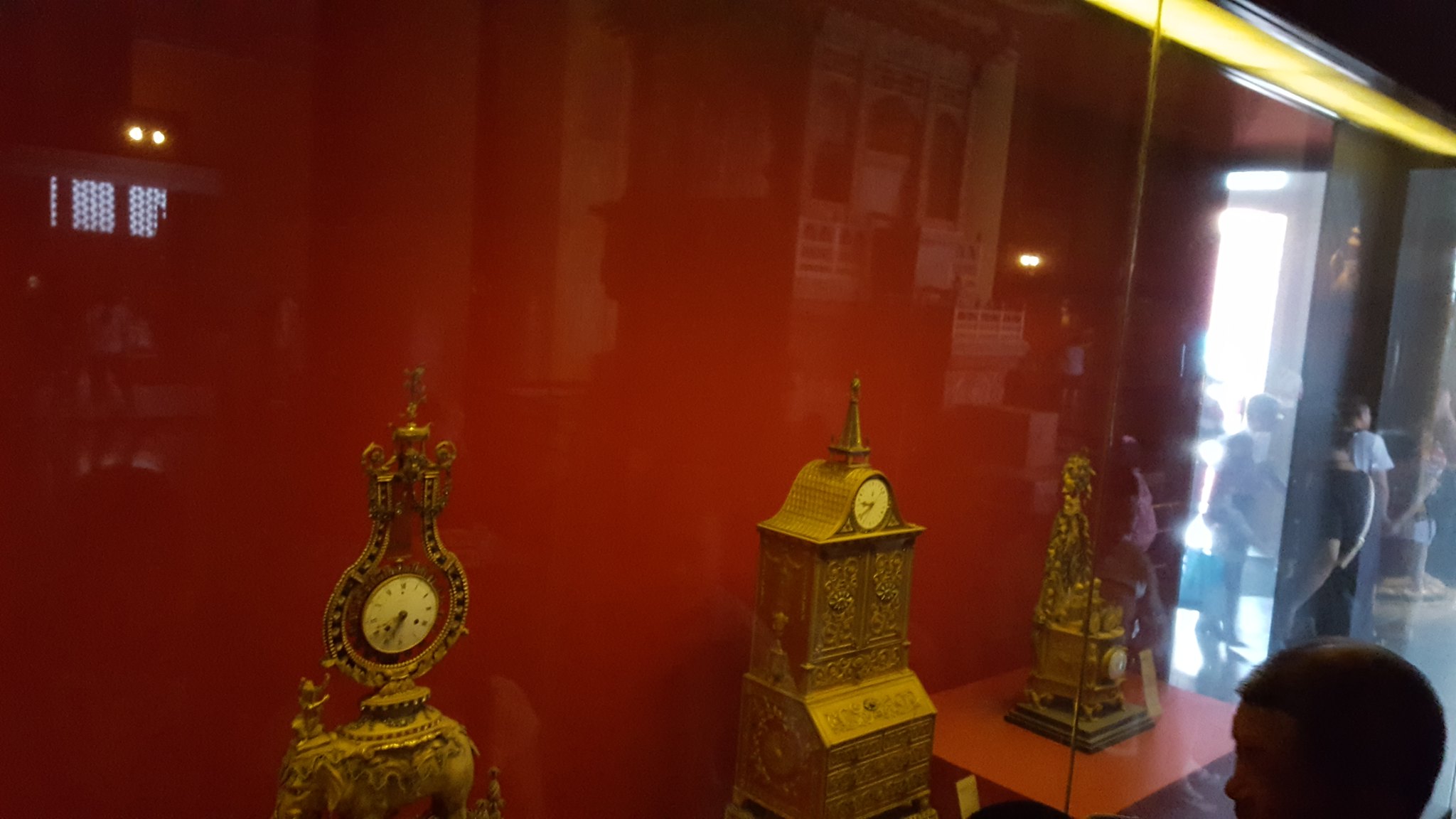The image features a display case within a museum, viewed from a slightly elevated angle. The case has a silver border and a yellow fluorescent light at the top, illuminating the contents. Reflections of people and lights from the room are visible on the glass panels of the case, making it hard to discern colors. Inside, a rich red background highlights three ornate golden antique clocks, each with intricately designed faces. The clock on the left is tall and slender, the center one is broad and almost as tall, while the one on the right is short and set on a red stand. In the lower right-hand corner, there is a silhouette of a young man's head, apparent from the mouth up, gazing at the display. The reflection on the right side of the image reveals a bright light and a person looking at something else, suggesting a busy museum environment. The overall scene captures a rich, historical ambiance through the gold, red, and reflective elements.